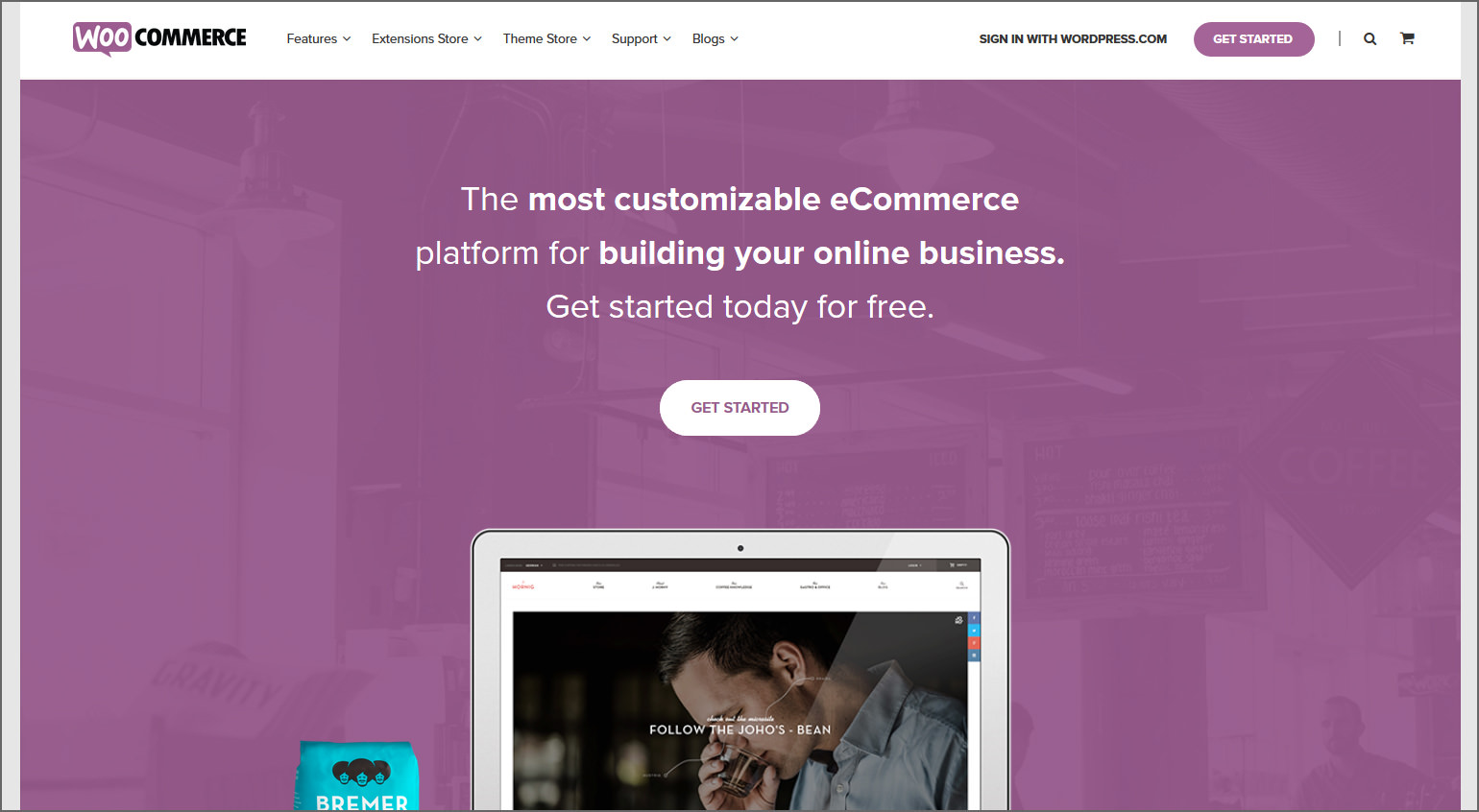This image is a screenshot from the WooCommerce website. It features the WooCommerce logo prominently centered at the top, with "Woo" displayed in a purple speech bubble and "Commerce" in black text. The website's navigation bar below the logo includes dropdown menus labeled Features, Store, Theme Store, Support, and Blogs. 

The upper right corner of the page has a white space area with options for users to "Sign in with WordPress.com" and a prominent purple "Get Started" button. Additionally, there are icons for a magnifying glass and a shopping cart.

The central section of the webpage has a light purplish, almost rose-colored background. In this section, bold white text states, "The most customizable eCommerce platform for building your online business." Below this text, a white button invites users to "Get started today for free." A smaller white button under the call-to-action text reads “Get Started.” The middle area also contains an illustrative image showing examples of websites and how they can be built using the WooCommerce platform.